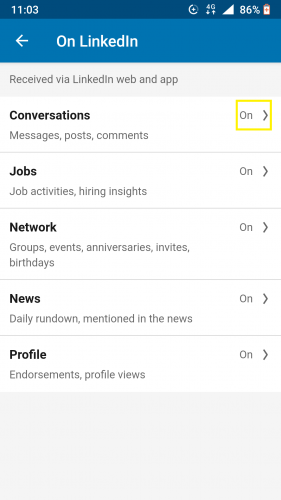This is a detailed screenshot of the LinkedIn settings page on a mobile device. At the top, there is a blue bar displaying "LinkedIn" in white text, accompanied by a white back arrow on the left. Below the blue bar, there is a gray section indicating "Received via LinkedIn web and app."

Five settings options are listed below this section, each within a white background. The titles of these settings are presented in bold black text, accompanied by regular gray text underneath them. The five categories are: Conversations, Jobs, Network, News, and Profile. Each setting row includes a toggle switch and a right-pointing arrow icon on the right side, and the rows are separated by thin dividing lines.